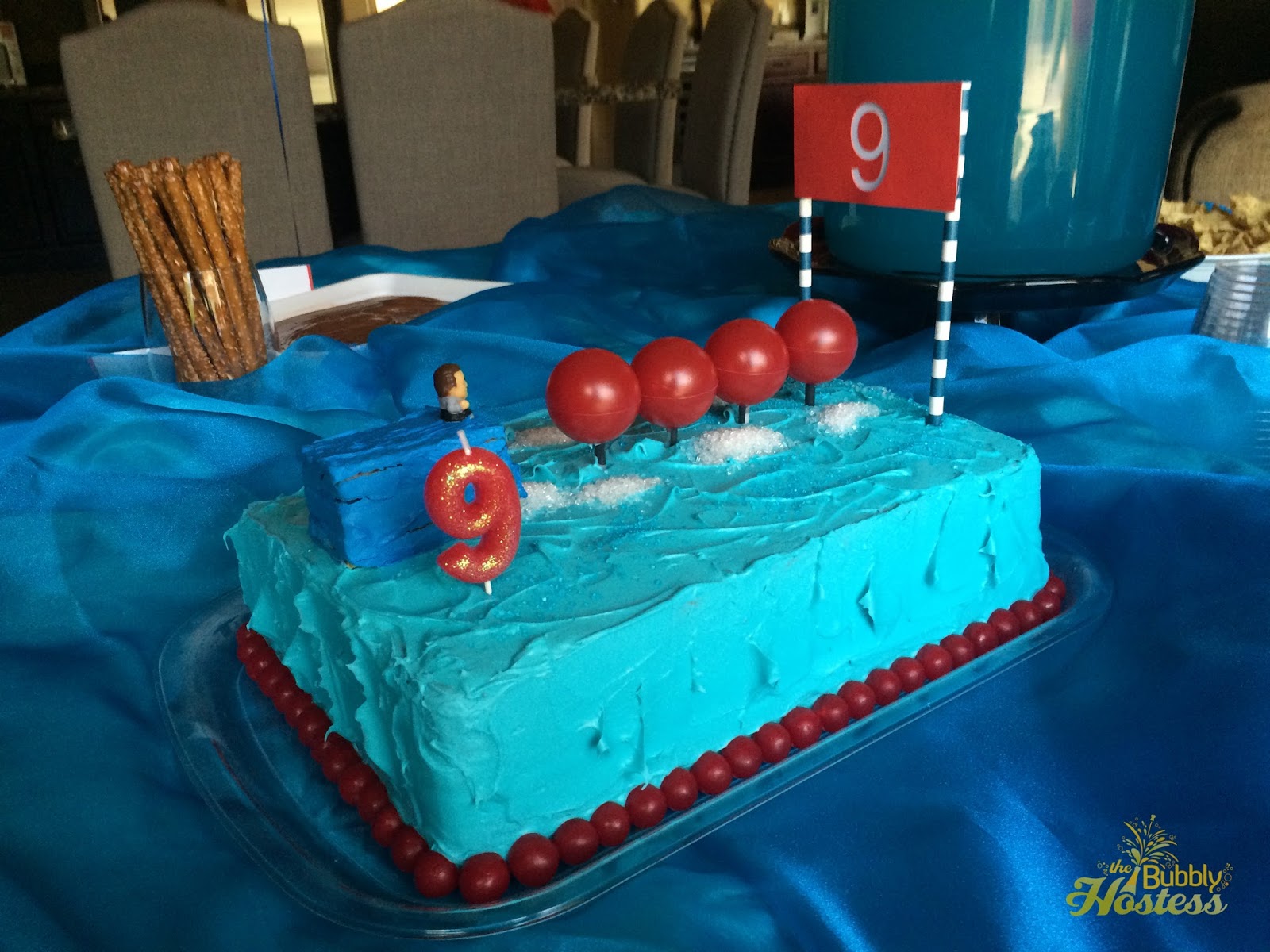The image presents a detailed scene centered around a homemade cake with a 'Wipeout' TV show theme, perfect for a nine-year-old's birthday celebration. The cake, adorned with blue buttercream icing, features a small character standing on a blue rectangular platform on the left side. A notable feature is a row of red balls resembling the iconic bouncing obstacles from the show, leading to a finish line marked by pirouette sticks and a red banner with a white number nine in its center. A red number nine candle is placed near the bottom left of the cake, surrounded by more red balls and white sprinkles. The cake sits atop a loosely scrunched blue satin tablecloth meant to mimic water. The backdrop includes additional elements: a pretzel stick-filled cup on the left, a plate with Nutella, and a glass jar filled with chocolate bars at the bottom right. The setting, color-coordinated in shades of blue, red, white, and brown, underscores the festive atmosphere, further highlighted by the text 'The Bubbly Hostess' visible in the bottom corner.